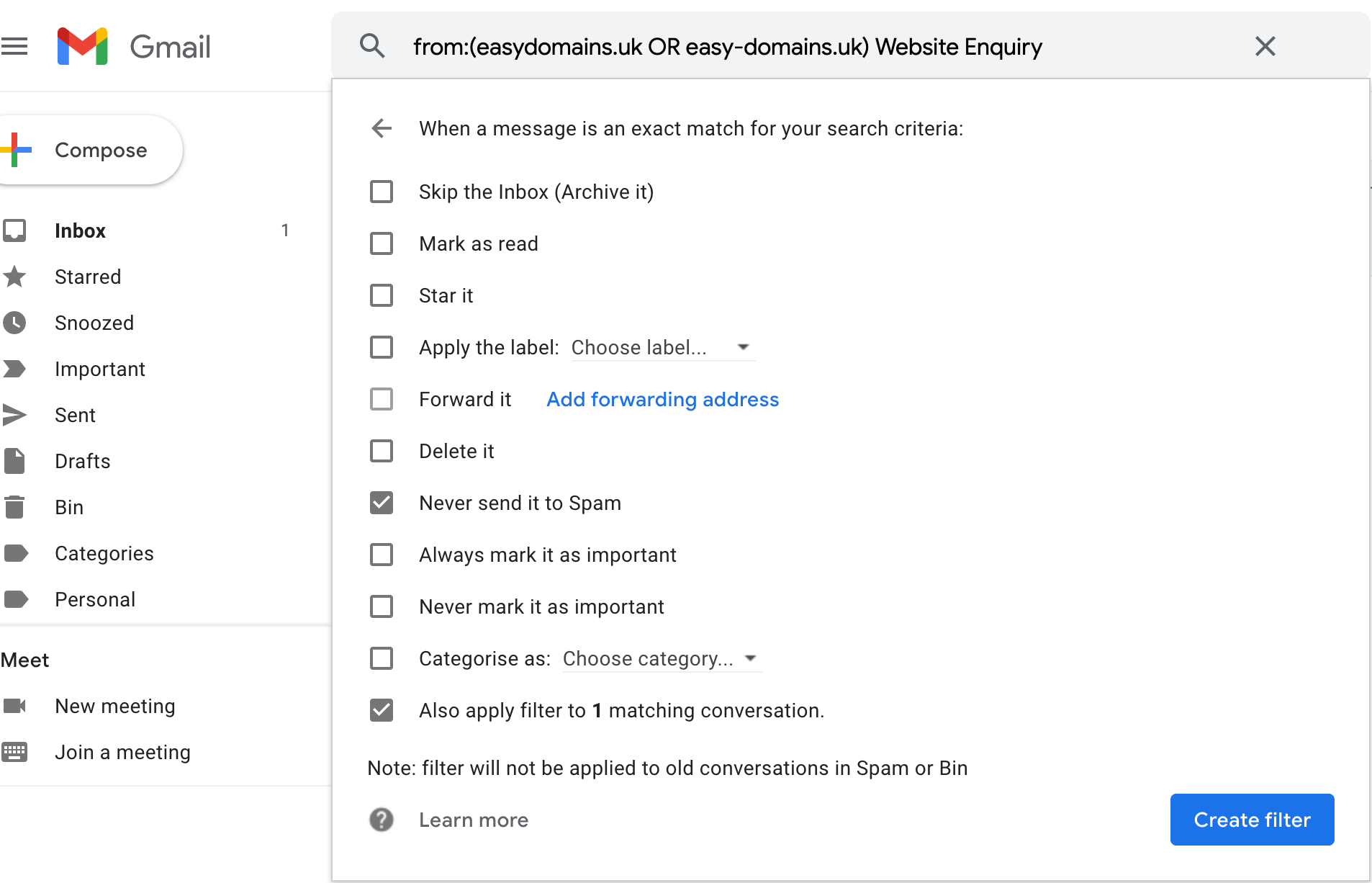This is an image of the Gmail interface. On the top left-hand side, we observe the "Gmail" label accompanied by the iconic "M" logo. Below this, a vertical navigation menu extends from top to bottom. The first element of this menu, situated between the logo and the vertical navigation, is the "Compose" button used for drafting new emails. As we proceed down the menu, the following labels appear in sequence: "Inbox," "Starred," "Snoozed," "Important," "Sent," "Drafts," "Bin," "Categories," and "Personal." Further down, there is a section titled "Meet," which includes the options "New Meeting" and "Join a Meeting."

Dominating the main content area is a search bar at the top, equipped with a magnifying glass icon. The search bar contains the text "From: Easy-Domains.uk (Website Inquiry)" as an example of a search result. Below this, there is a note indicating that the message is an exact match for the provided search criteria.